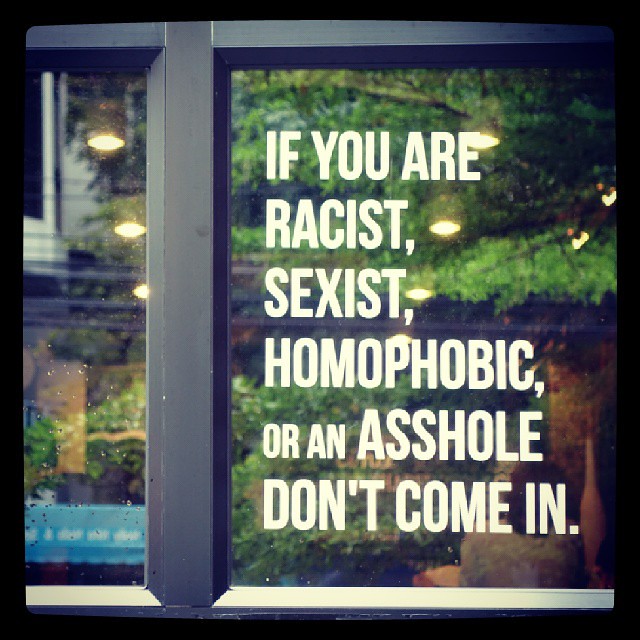The image depicts a digitally generated close-up of a storefront window with a black frame. The glass window features grey borders and prominent white text in capitalized, bold letters stating, "IF YOU ARE RACIST, SEXIST, HOMOPHOBIC, OR AN ASSHOLE, DON'T COME IN." This bold statement is the primary focus of the image. The windowpane reflects green trees and the street behind the photographer, including a blue awning and a brick-colored building. Tiny droplets of water or condensation are visible on the glass. Behind the window, interior lights and part of a house with windows suggest the setting is a garden or backyard area.